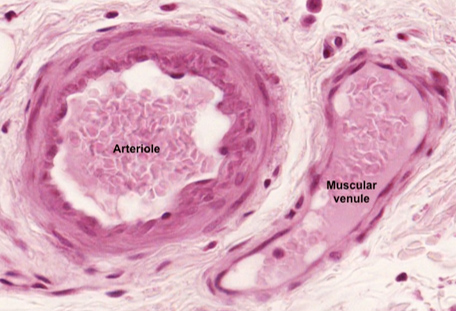The image appears to be a detailed digital drawing focused on health-related content, likely sourced from a medical site or used for educational purposes. On the left side of the image, there's a circular depiction in shades of pink and white, labeled "Areola" in black text. This area features varying hues of pink and lighter pinks. On the right side, the image showcases a longer, island-like structure labeled "Muscular Venule." The background surrounding these structures is predominantly white, interspersed with small red and pink dots, adding to the intricate detailing of the image. The illustration seems to represent microscopic views of specific body parts or cells, providing a visual reference that might aid in understanding certain medical conditions or anatomical features.